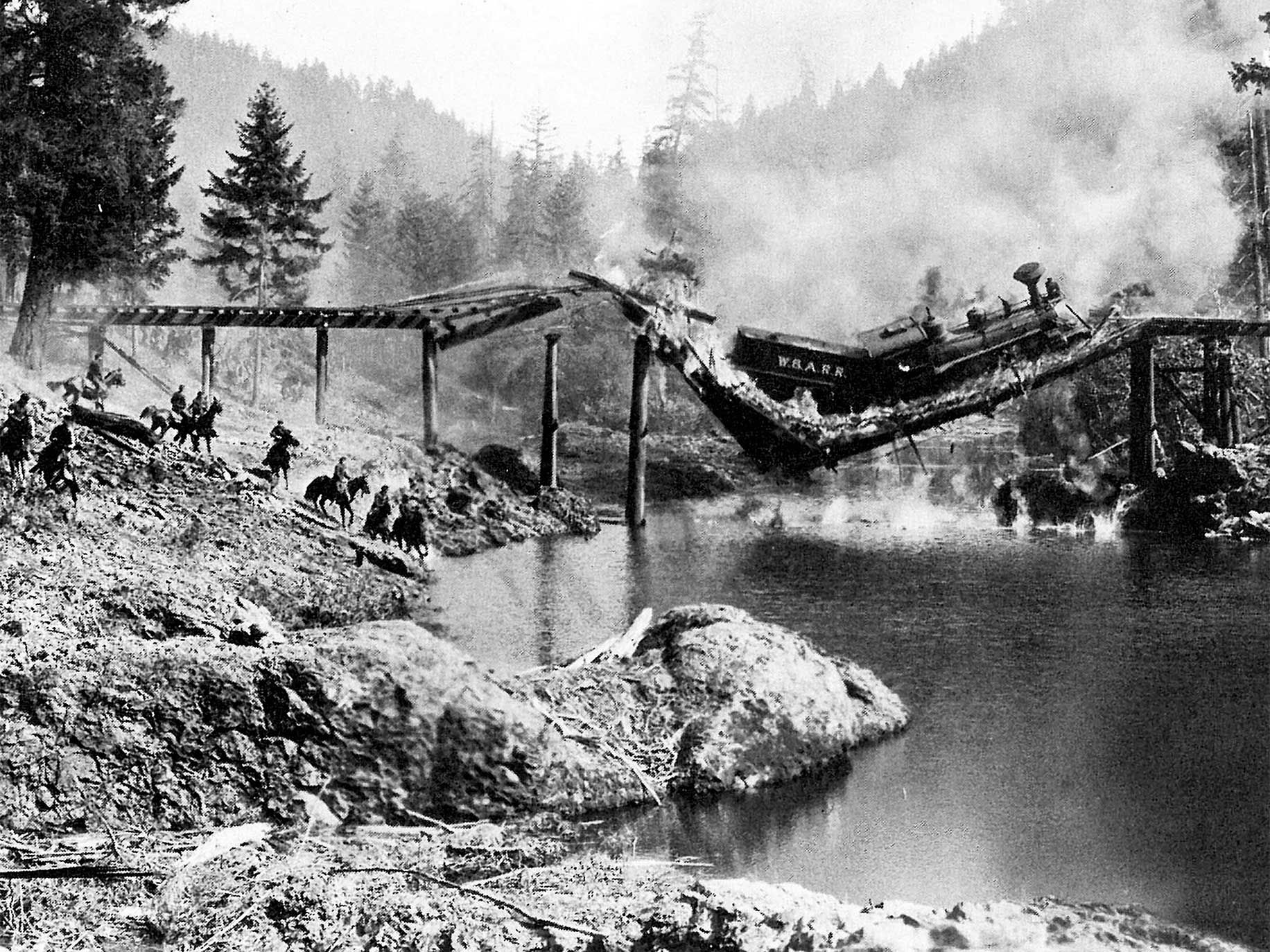This black-and-white photograph, likely from the late 19th or early 20th century, captures a dramatic train wreck over a river, possibly in the Pacific Northwest. The scene is dominated by a damaged wooden railroad bridge, its collapse causing a large black locomotive and its coal car to plunge towards the water below. The area is shrouded in thick fog, adding a somber mood to the chaotic event. In the background, tall evergreens and mountainous terrain frame the disaster. Several men on horseback are present, seemingly assessing the situation or searching for survivors amidst the wreckage.